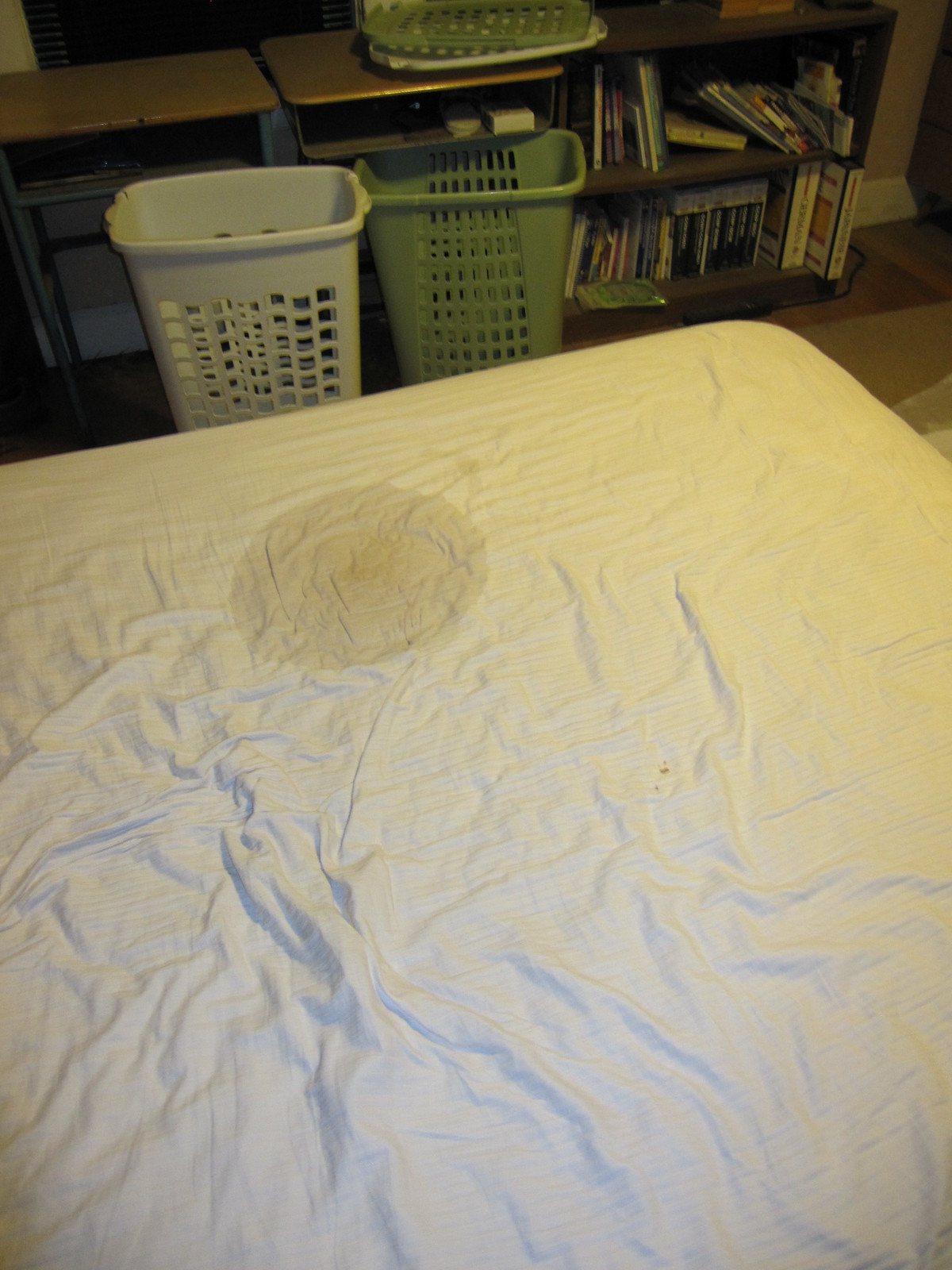In this photograph of a bedroom, the focal point is a king-size mattress, stripped down to a wrinkled white bottom sheet with faint light blue stripes. Prominently visible on the sheet is a circular stain with a brownish, wet appearance and a yellowish center. Surrounding the bed are multiple pieces of furniture and laundry baskets. In front of the bed, on a hardwood floor partially covered by a rug, lie two plastic laundry hampers—one green and one white. An additional green laundry basket is placed on one of the two standard desks to the left side of the bed, which feature shelves underneath them for storage. To the right, there's a bookcase packed with numerous books. The room is painted brown with white molding at the bottom, adding a residential ambience. Overall, the image captures a somewhat cluttered and lived-in bedroom scene marked by the prominent wet stain on the bed.